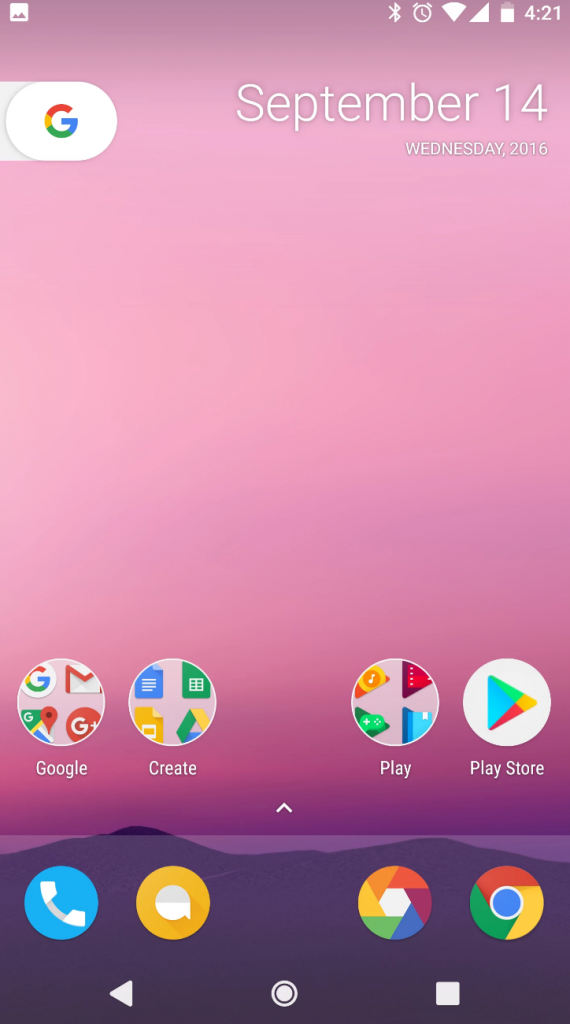This is a detailed description of a mobile phone screenshot. The image is vertically oriented and features a gradient background that transitions from a purplish pink at the top to a lighter rose color at the bottom. At the very bottom of the image, there appears to be a vague, abstract design depicting mountains and possibly a sea.

The screenshot was taken at 4:21, as indicated by the time in the top right corner. Additional icons include an alarm clock, Bluetooth, and a battery level showing approximately 75% charge. The date displayed is Wednesday, September 14, 2016.

At the bottom of the screen, there are eight circular icons grouped in pairs. From left to right, these include:

1. Google apps: Gmail and Maps
2. Google Plus
3. Create suite: Sheets and a word processor
4. Google Drive
5. Play Store

Below these groups, there are icons for phone calls, texting, an unidentified application, and Google Chrome.